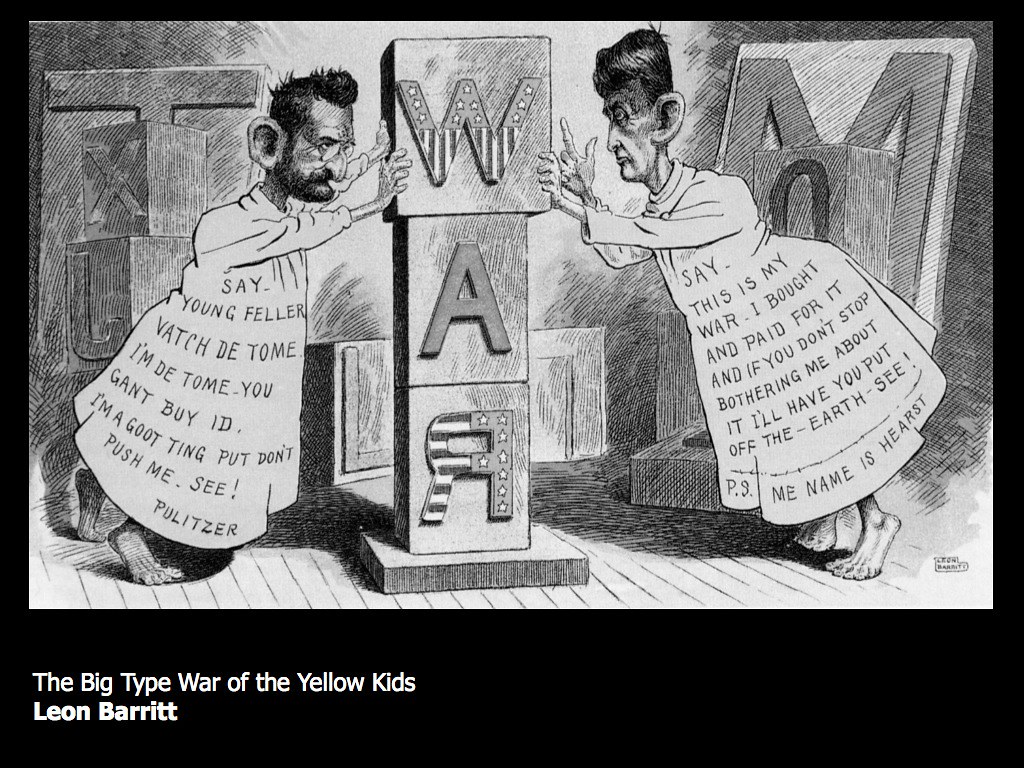This detailed black-and-white political cartoon by Leon Barrett, titled "The Big Type War of the Yellow Kids," is meticulously illustrated in pencil. Central to the composition are three stacked blocks that spell out the word "WAR," with the "W" at the top, "A" in the middle, and a backwards "R" at the bottom, both the "W" and "R" adorned with American flag patterns. Flanking these blocks are two men, each pushing against them. 

On the left, a bearded man with glasses wears a white dress inscribed with, "Say young feller, watch de tome, I'm de tome, you can't buy I.D. I'm a good ting, but don't push me — C. Pulitzer." On the right, another man with black hair, similarly attired, has the text on his dress reading, "Say, this is my war, I bought and paid for it, and if you don't stop bothering me about it, I'll have to put off the earth — C.P.S., my name is Hurst."

In the background, more blocks and letters are visible, hinting at the chaotic nature of the argument. The entire scene is enclosed by a black outline, with a whiter section at the bottom. The cartoon's caption, "The Big Type War of the Yellow Kids," is prominently featured below the illustration.